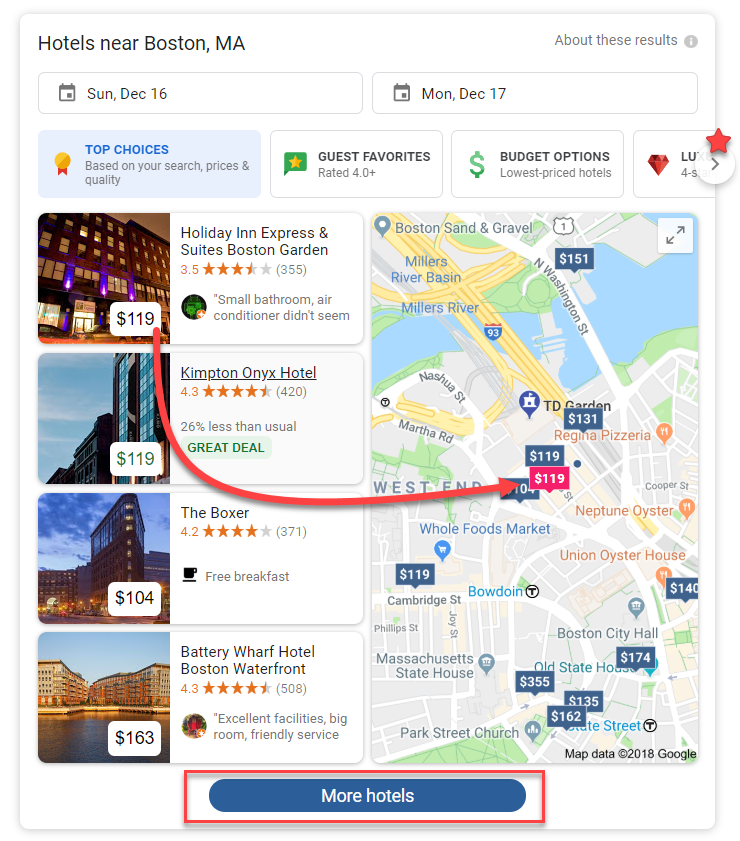A mobile app displaying hotel options near Boston, MA, is on the screen. The app appears to be similar to Trivago, Travelocity, or Hotels.com. The search results are for hotels available from Sunday, December 16th to Monday, December 17th. The app highlights several options under categories such as "Top Choices", "Guest Favorites", and "Budget Options". 

In the search results, the Holiday Inn Express & Suites Boston Garden is prominently featured with an arrow pointing to its location on a map. It's priced at $119 per night. The map, marked with a red box around "More Hotels", shows several other hotels including Kimpton Onyx Hotel, The Boxer, and Battery Wharf Hotel Boston Waterfront. Each hotel listing includes gold stars indicating their review ratings and the total number of reviews. For instance, the Kimpton Onyx Hotel has a "Great Deal" label in a green box. 

At the bottom right corner of the map, there is a star icon and the text "Map data © Google".